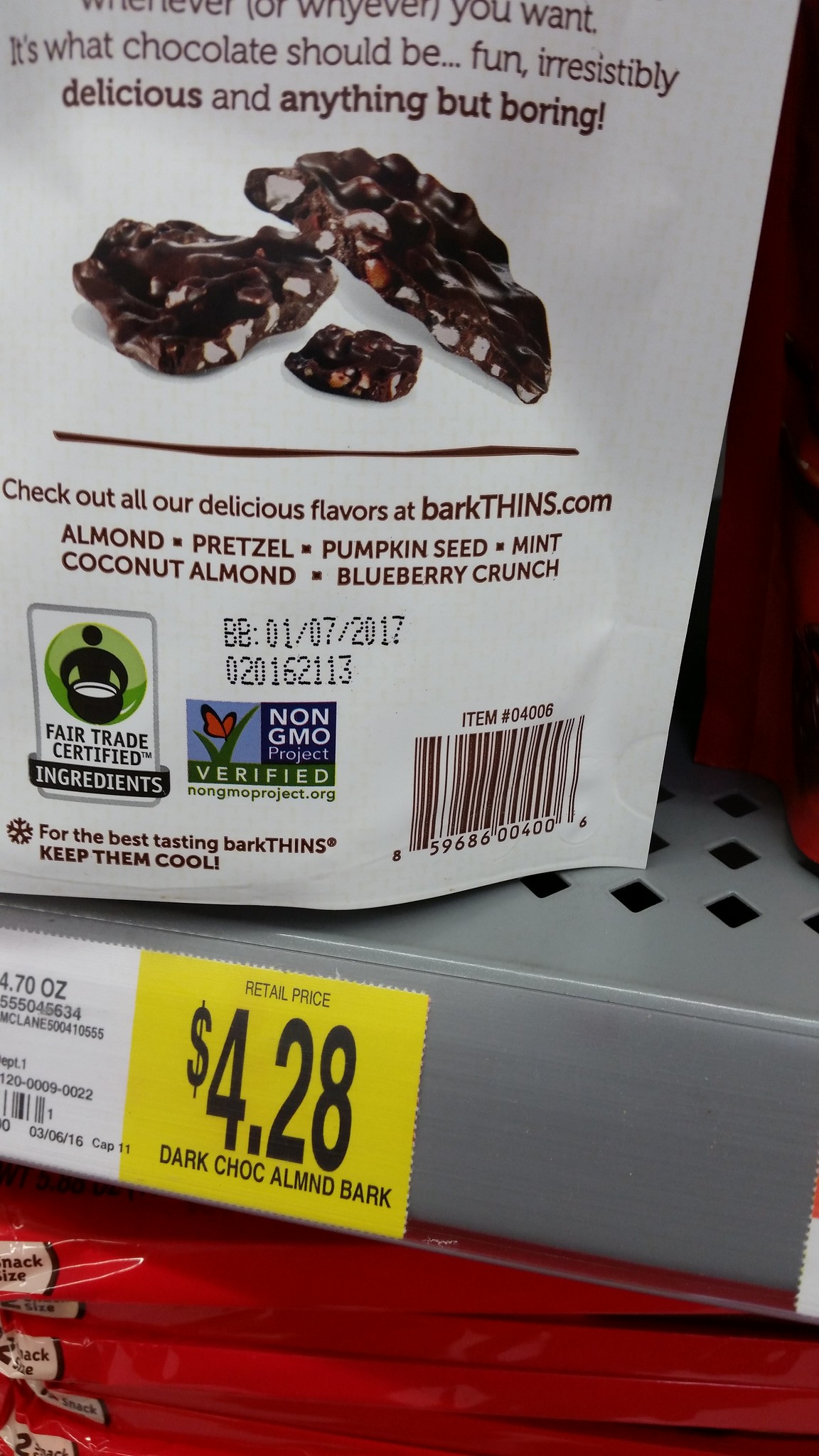A box of pretzel snacks is prominently displayed on a metal store shelf with distinctive square designs. The box, which occupies the upper left corner and extends to the middle of the image, is slightly tilted, providing a clear view of its branding and artwork. To the right of the pretzel box, another food item is partially visible, resting on the same shelf. A price tag placed below reads "$4.28" and describes the item as "Dark Chalk Almond Bark."